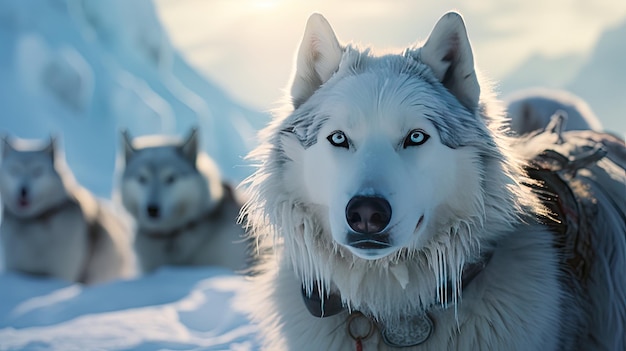The image features a close-up of a striking white dog, likely a husky or wolf, set against a snowy, outdoor background that includes blurred snow-covered mountains and hills. The dog, situated on the right, has icy blue eyes with black pupils and appears to have wet fur, with some tufts hanging down, suggesting it has been in the snow. It wears a strange collar and possibly a harness or blanket on its back. The dog's fur has hints of gray and blue, and its ears stand upright with a hint of pink. Behind this central animal, to the left, are two more similarly bred dogs, though they are blurred due to the depth of field. The background is bright with visible sunlight, indicating daytime, and the scene is coated in thick snow. The atmosphere conveys a cold, wintry environment, possibly suggesting the dogs are part of a sled team or a pack acclimated to such harsh conditions.